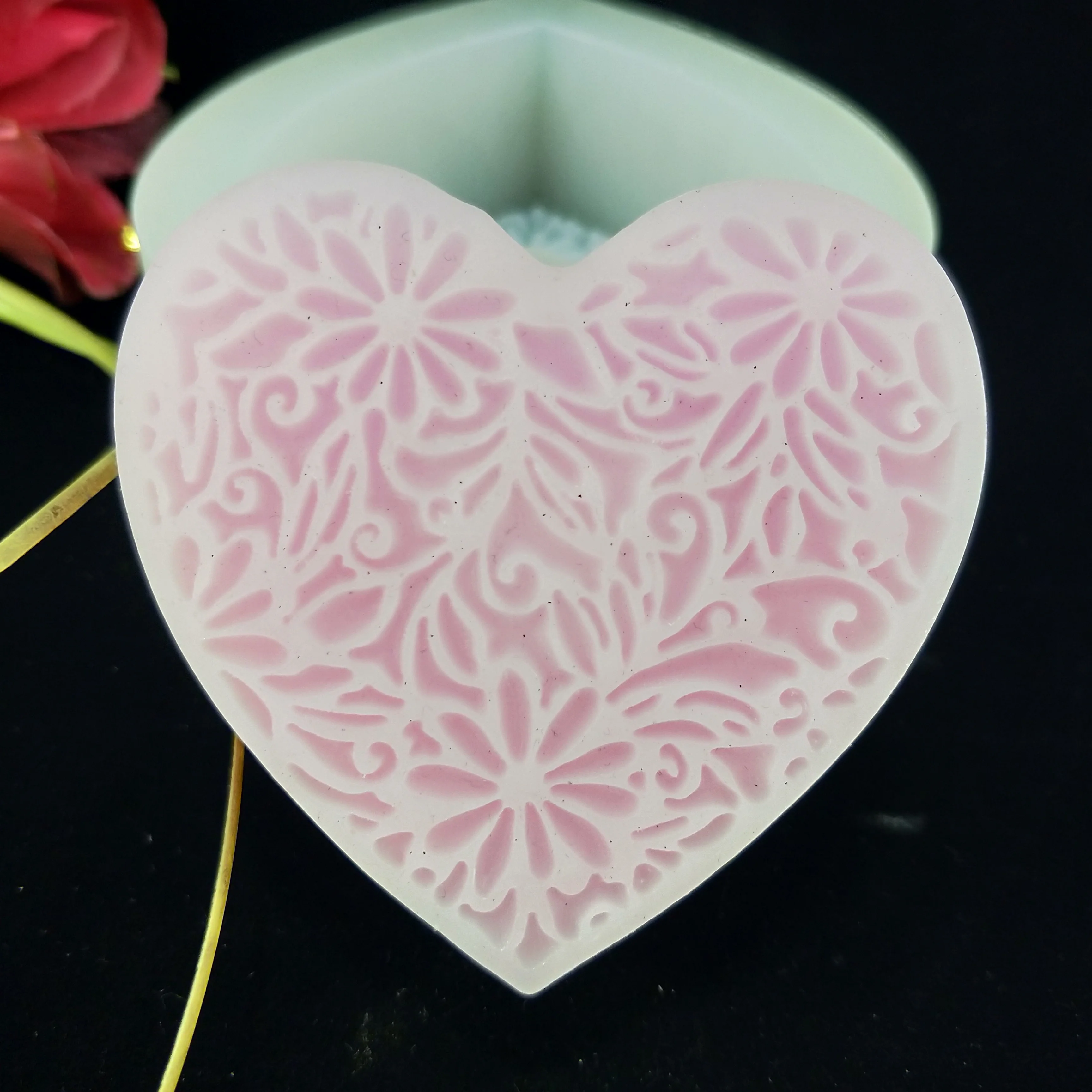In the image, a delicately crafted heart-shaped object, potentially a bar of soap or a wax decoration, showcases intricately carved floral patterns filled with vibrant pink color. The base material of the heart appears to be a soft, whitish pink hue. Behind the heart, a mold used for shaping it is partially visible, subtly detailed by a corner showing the heart-shaped bottom. The heart rests on a black surface, giving the entire setup a striking contrast.

To the left of the heart, red fake flower petals, accompanied by green stems, partially enter the frame, adding a touch of natural elegance. Additionally, a thick golden string or thread is noticeable on the left side of the image. The background includes a mint green object, possibly a candle or soap holder, providing an appealing hue juxtaposition. The heart itself features small black speckles, suggesting it might be crafted with natural ingredients. The entire scene is bathed in soft shadows, accentuating the intricate details and enhancing the overall visual appeal.